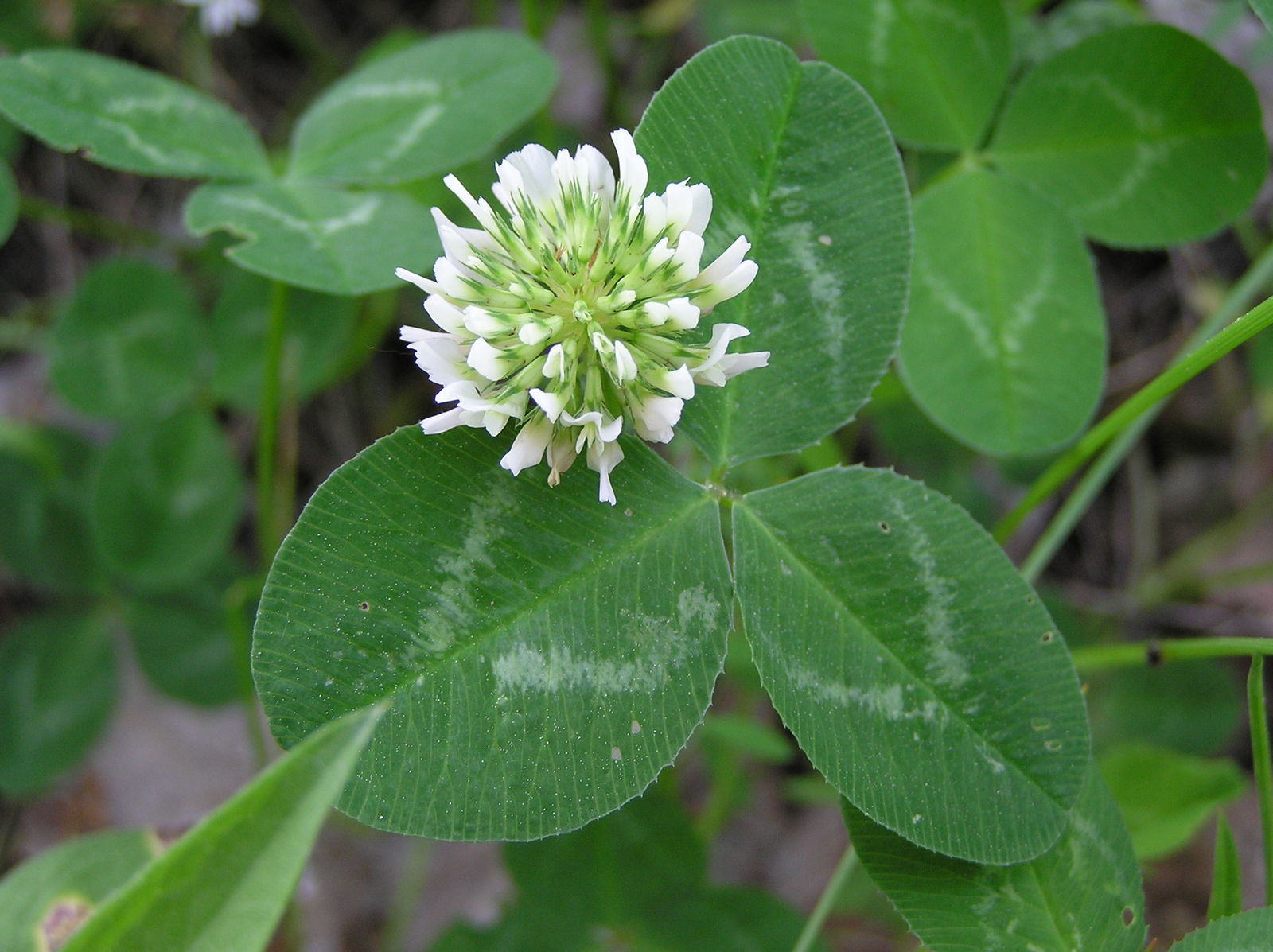This detailed, close-up photograph features a vibrant three-leaf clover in full bloom. Dominating the center is a striking white clover flower, presented in a starburst pattern. From its light green center radiate slender green stems, each culminating in a small, delicate white flower. Extruding as a cluster, the flower creates an impression of a starburst dome with around 20 to 40 tiny blossoms. The surrounding environment, though blurred, reveals a few other distant clovers, some grass, and the ground, faintly visible. The image seems to have been captured on an overcast day, lending a soft, muted quality to the colors and contrast. In the background, out-of-focus brown stems or branches, other green leaves, and a notable leaf with a brown spot add depth to the natural setting. Visible as well is a three-leaf cluster with a distinct pale whitish-tan vein running across each leaflet, highlighting the intricate details of the clover plant.